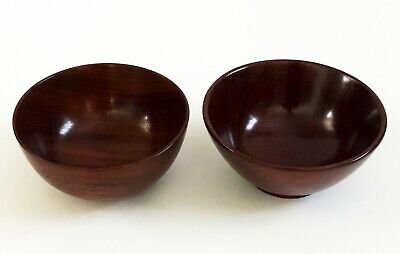This close-up image features two dark brown wooden bowls, positioned side-by-side on a white background or tabletop. The photograph appears to be taken at a slight angle from above, allowing visibility into the empty bowls. Both bowls are made of polished wood, showcasing a glossy finish that highlights their fine grain. The bowl on the left is perfectly round, resembling a half-circle, while the bowl on the right has a distinct shape with a smaller base and tapered sides, giving it a more triangular appearance. This polished, high-quality craftsmanship and the minimalistic design suggest that the bowls might be part of a collection, potentially aimed for a sale listing, similar to what might be seen on eBay.